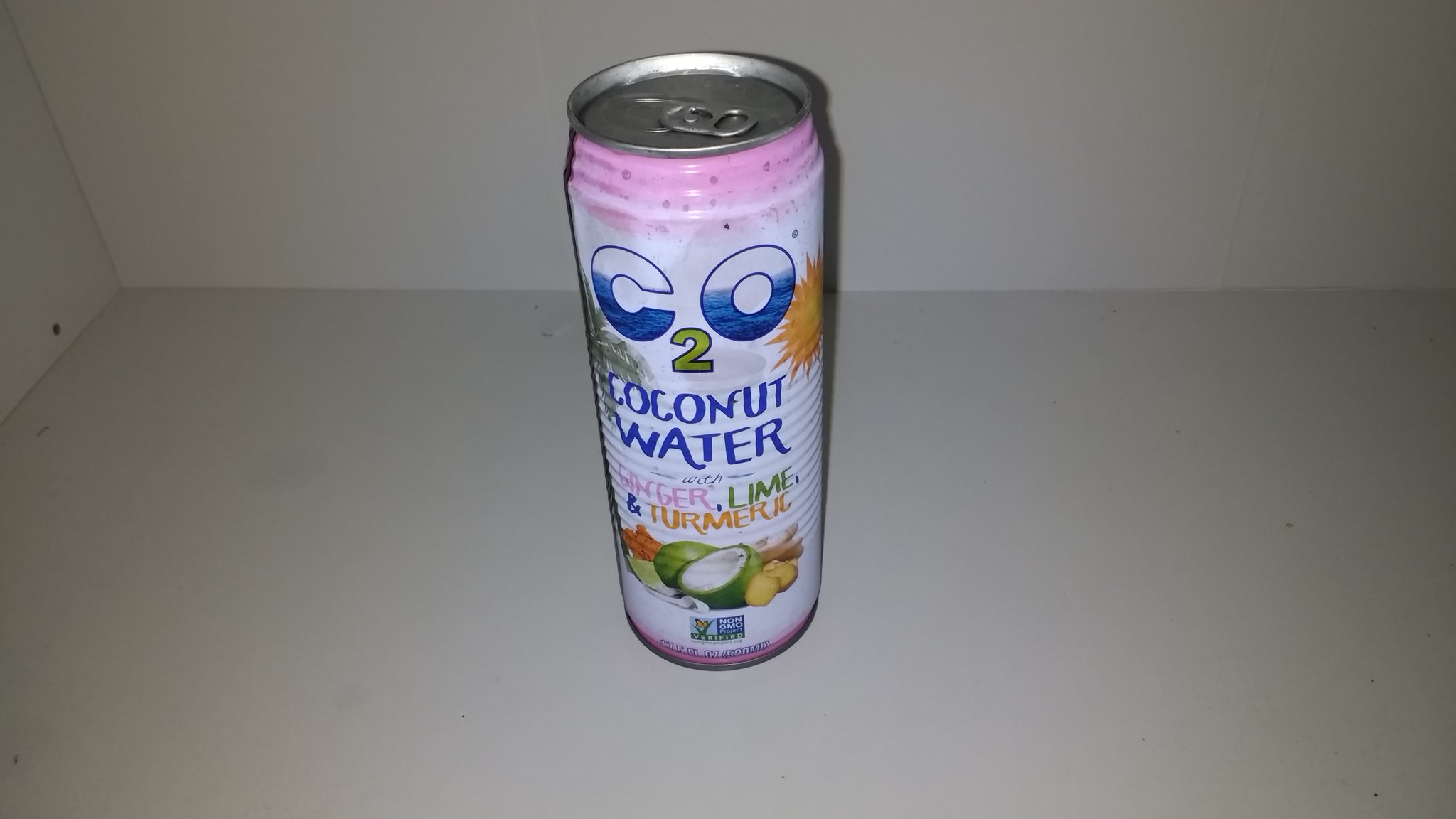Photograph depicting a 12 oz can of C2O Coconut Water with Ginger, Lime, and Turmeric flavoring, placed against the backdrop of a pristine white room or cupboard. The can features a predominantly white design accented with splashes of pink and vibrant graphics of ginger, lime, and turmeric around its center. Notable elements include the "C2O" text incorporated with imagery of an ocean, sun, and palm tree within the letters 'C' and 'O'. Additionally, a "Non-GMO Project Verified" sign is prominently displayed, emphasizing the product's quality. The can's sleek, tall, and lean shape stands out in the minimalist setting.